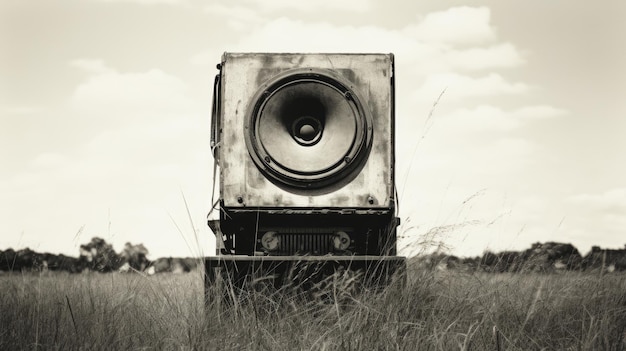The black and white photograph captures a vintage, distressed, and worn-out retro speaker with a distinct box-like, square structure. This old-style speaker, featuring a centrally placed circular woofer, stands on a rectangular base situated in the middle of an expansive, grassy field that appears greyish, reminiscent of dried hay. The scene is enveloped by a vast sky with light grey tones and scattered white clouds. In the background, a line of dark grey trees creates a lush horizon. The overall setting evokes the ambiance of retro musical instruments or appliances, with the speaker dominating the foreground, looking neglected yet enigmatic in its solitude amidst nature.